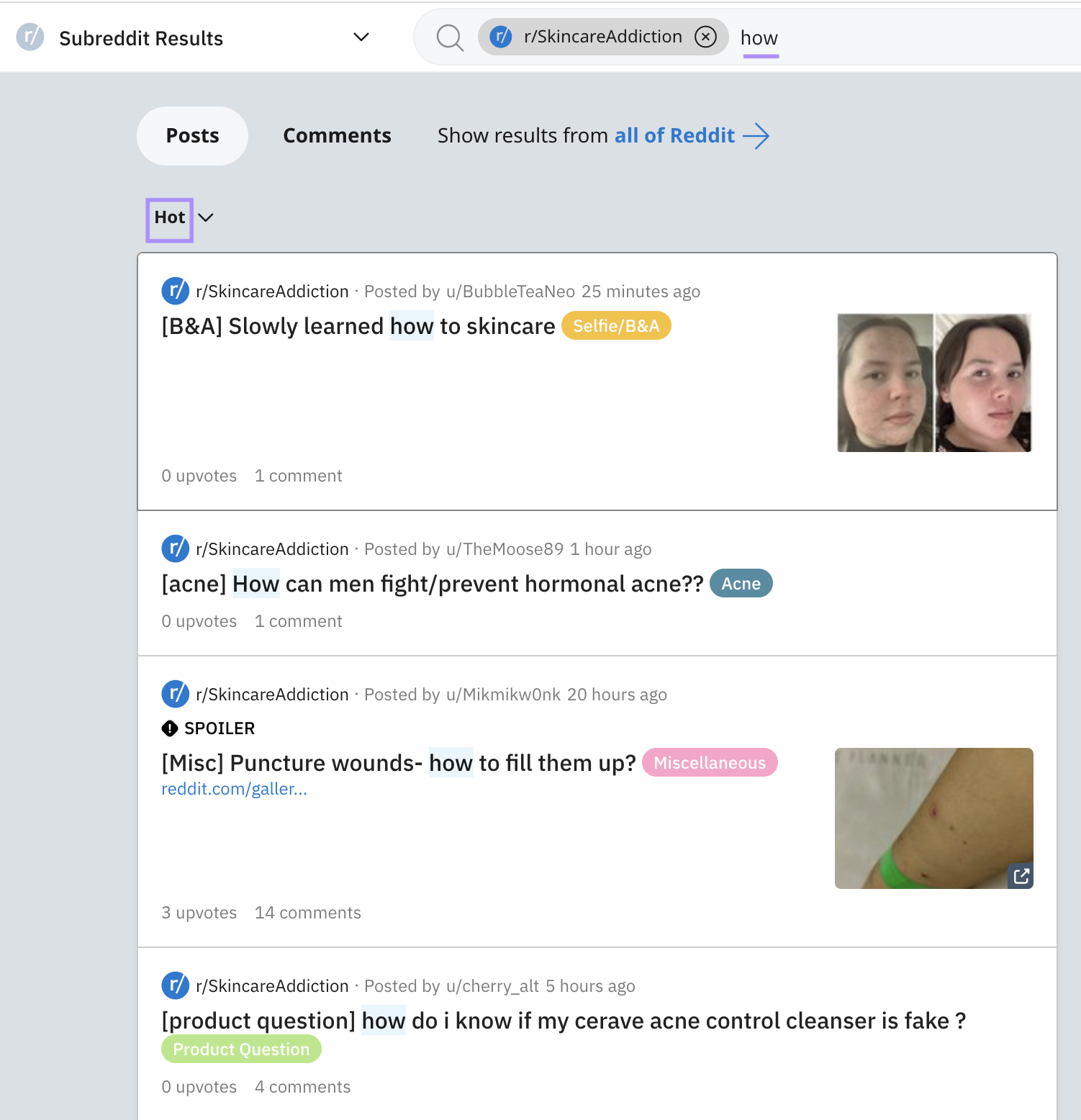In this image, a search on Reddit is performed within the "SkincareAddiction" subreddit. The search bar located at the top features a magnifying glass icon and contains the text "r/SkincareAddiction," indicating that the search is specific to this subforum. To the right of the search bar, the word "How" is underlined in purple. Below the search bar, various search results are displayed sequentially. These include posts, comments, and an option to show results from the entirety of Reddit, focusing specifically on the topic of skincare.

The top left section of the screen displays a list of subreddit results, accompanied by a dropdown arrow for further navigation. The search returns several specific posts, beginning with "Slowly learned how to skincare Selfie/B&A," followed by "Acne: How can men fight or prevent hormonal acne?" Another result is marked with a spoiler warning, addressing "Puncture wounds: How to fill them up, miscellaneous." The final result is a product inquiry, asking "How do I know if my keratin acne control cleanser is fake?"

Each post pertains to common issues and questions within the skincare community, reflecting the diverse concerns and advice-seeking behavior of users within the "SkincareAddiction" subreddit.